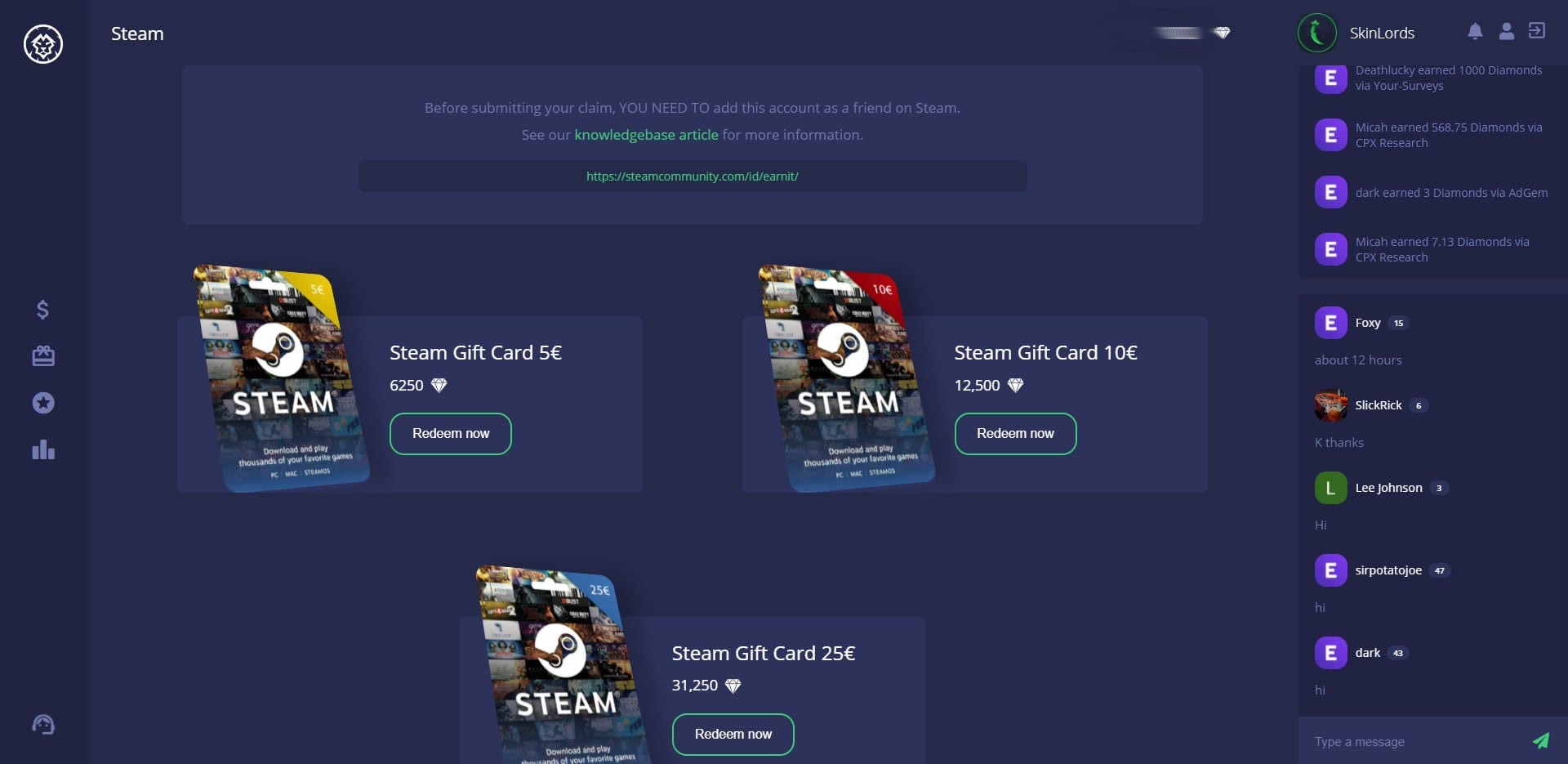A screen capture of a website selling Steam gift cards is displayed, specifically showcasing the official Steam platform dedicated to gaming enthusiasts. The interface prominently advertises Steam gift cards available in three denominations: 5 euros, 10 euros, and 25 euros. Each gift card is visually distinguished by different colored corners—green for the 5-euro card, red for the 10-euro card, and blue for the 25-euro card. The design on each card features a collage of tiny game images along with the prominent Steam logo. To the side, a navigation panel includes various tabs labeled with different letters, potentially leading to other categories or sections of the website. The overall layout is user-friendly, emphasizing the ease of selecting and purchasing gift cards in various amounts.